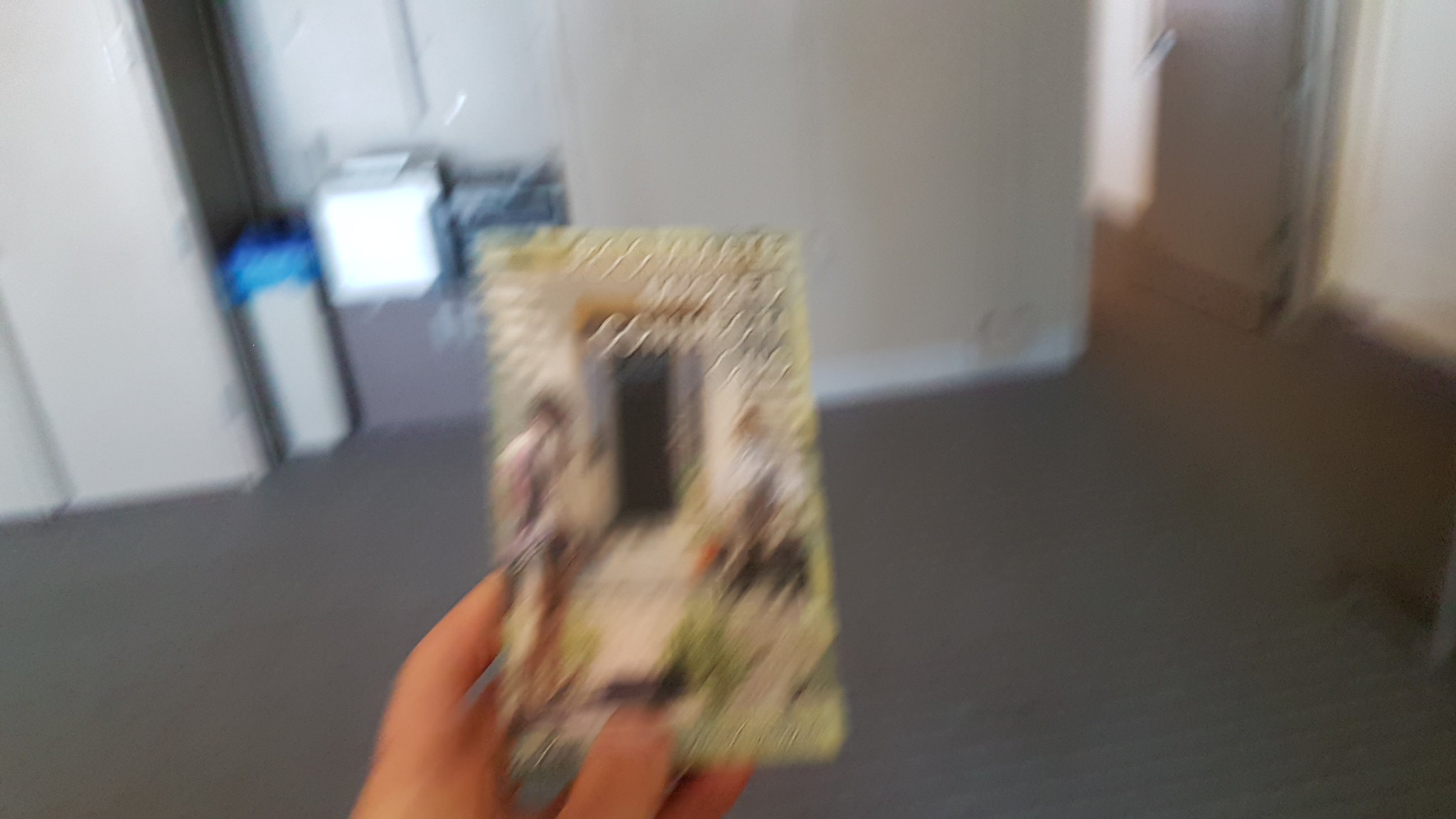The image features a blurry interior scene dominated by a large expanse of dark grey flooring. On the far side, a wall with a doorway is visible, surrounded by several indistinguishable objects, one of which may be a bin with a blue top. In the foreground, a partial hand is holding a picture, equally blurry. Upon close inspection, the picture seems to depict two individuals, one on the left appearing faintly male and another on the right possibly female. They are outdoors, standing in front of a doorway. However, the details remain unclear due to the overall blurriness of the photograph.